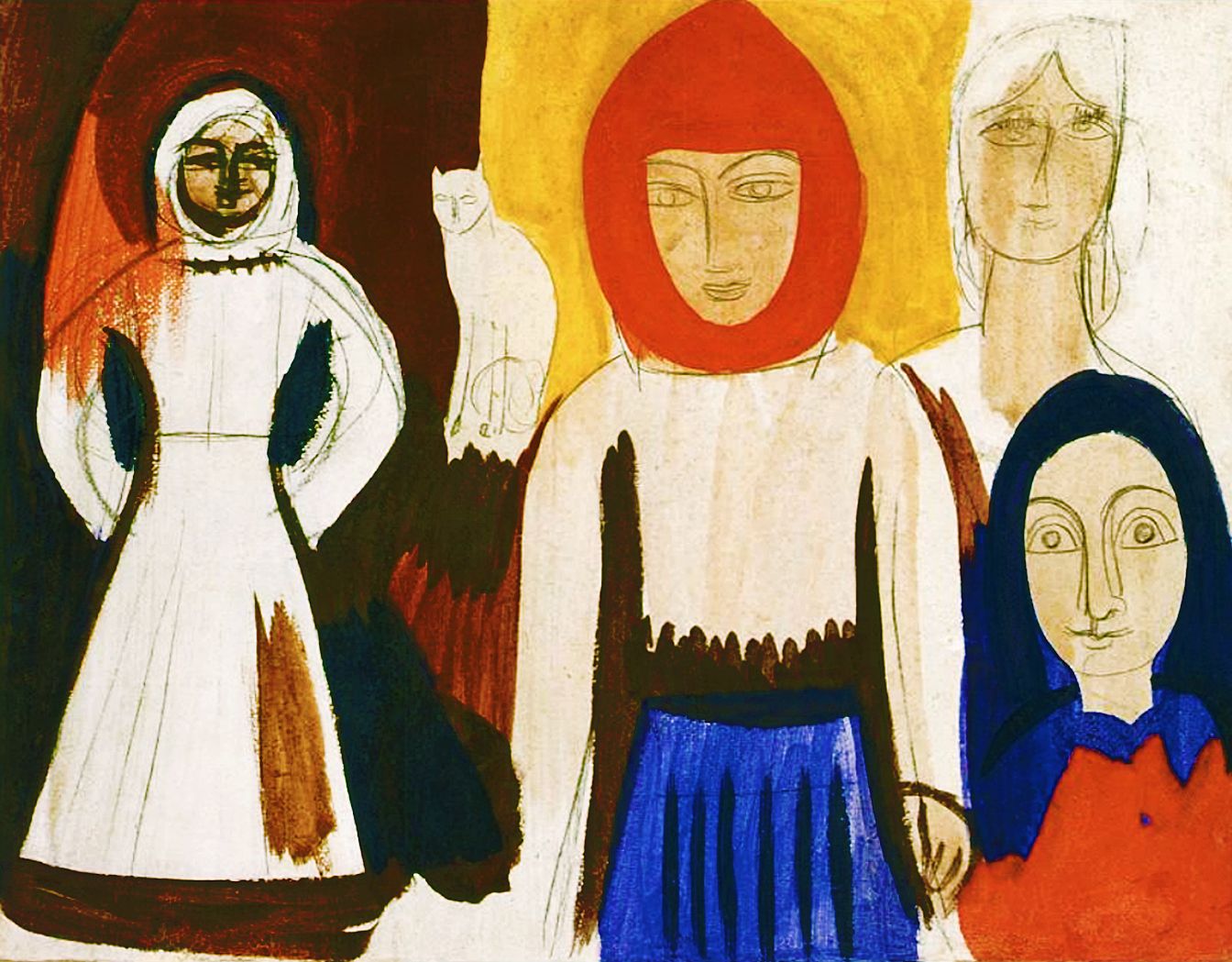In this very simple and minimalist painting, the artist uses crude and rudimentary lines, resembling an elementary school sketch. The image portrays four people and a cat, all facing the viewer, with each figure rendered in solid colors with minimal details and disproportionate features. 

From left to right, the first figure is a woman in a white dress, standing with her hands on her hips in a Superman pose and smiling. Next to her, towards the center of the image, there is a person wearing a long white shirt, a blue dress, and a red headgear encircling their head. Just to the right of this central figure is the silhouette of a white cat, positioned about two-thirds up the image, looking towards the viewer.

Further to the right, there are two more people depicted in a staggered manner. The front figure on the lower right has long blue hair and is dressed in a red shirt with a blue collar. Behind this character stands another person with long white hair, clothed in a white shirt. The overall scene is rendered with very basic, almost child-like, facial features and shapes, emphasizing simplicity and minimalism.